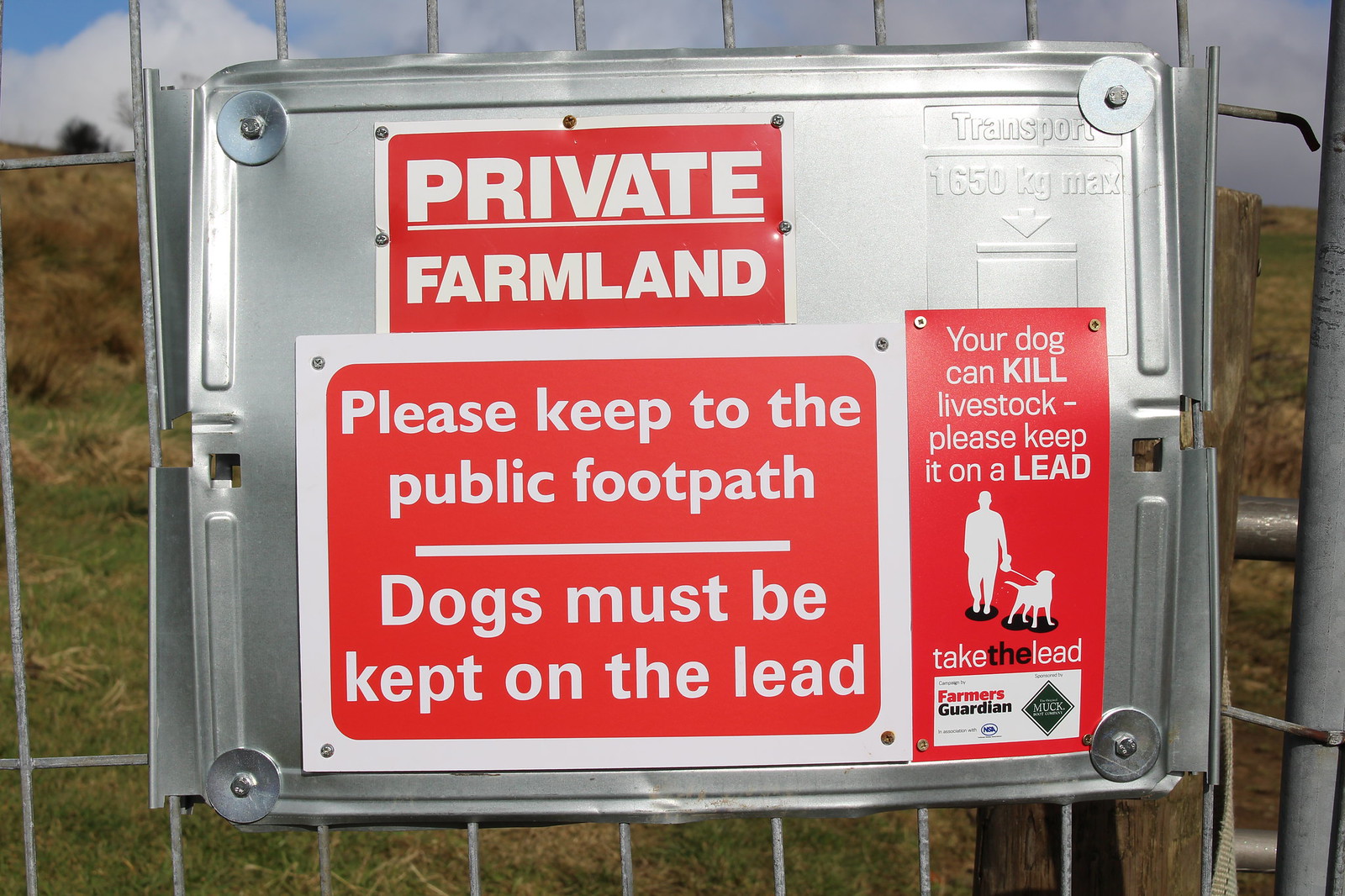In the foreground, a close-up of a metal aluminum sign hangs on a wire fence, which forms a part of a farmland boundary. The fence is composed of horizontal and vertical silver bars, and beyond it, tall grass and shrubs are visible. The central sign features several red placards, each with white text and riveted to the metal surface. At the top, one placard reads "Private Farmland." Below that, another sign states, "Please keep to the public footpath. Dogs must be kept on a lead." On the right side of the sign, a third placard warns, "Your dog can kill livestock. Please keep it on a lead," accompanied by an illustration of a person walking a dog on a leash. The detailed layout and clear instructions emphasize the importance of adhering to farm rules for public safety and the protection of livestock.